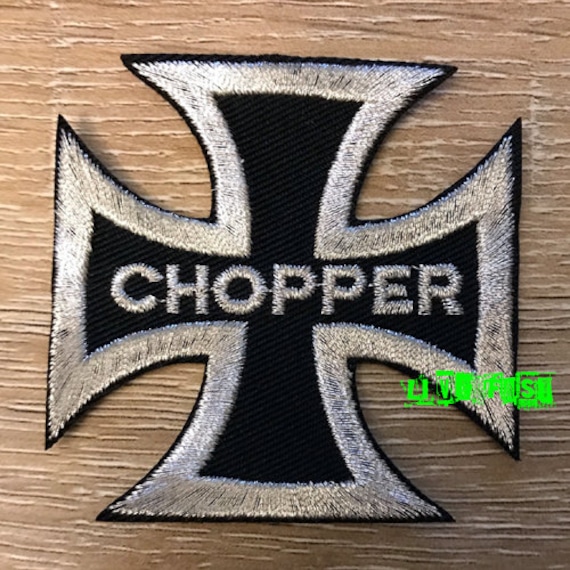The image displays a square patch, set against a wooden background, designed in the shape of an angular, flared cross, reminiscent of early 2000s motorcycle style. The patch has a black background with white embroidered borders. Centrally, in white embroidered text, the word "CHOPPER" is prominently featured. Additionally, there is some unclear bright green text at the bottom right point of the cross, appearing either in a foreign script or possibly an artifact of the image, which could suggest a company logo or branding. This patch, likely for a motorcycle club or gang, is designed to be sewn or ironed onto jackets, backpacks, or other items, serving as both a souvenir and a piece of biker identity.